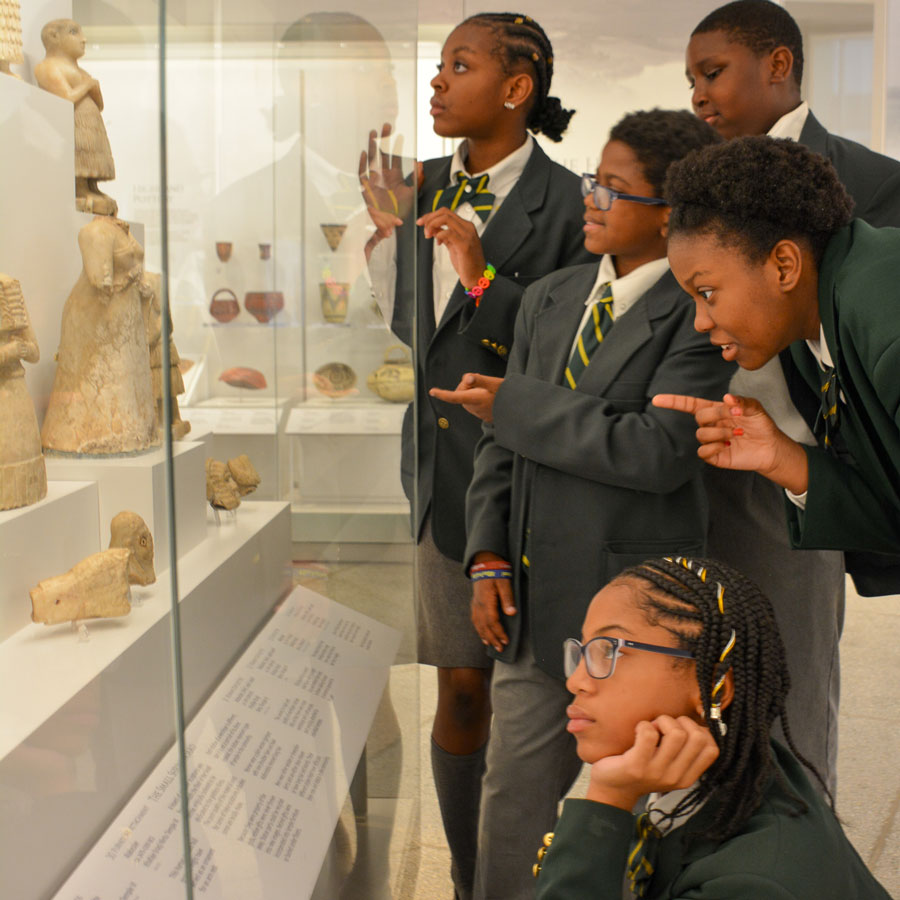The photograph captures five African-American school-aged children, three girls and two boys, dressed in dark gray blazers and light gray pants or skirts, each accessorized with gray and yellow striped or bow ties, standing in front of a glass case at a museum. The children are inspecting a collection of ancient, beige to brown-colored artifacts, such as pottery, figurines, or small statues, most of which are no taller than a foot. One girl with braided hair, adorned with yellow and white beads, kneels at the front, looking a bit bored with her hand under her chin. The rest of the children show varying levels of interest, with two wearing glasses and pointing at the display, while another boy stands slightly detached in the back. Additional display cases filled with similar artifacts can be seen in the background.